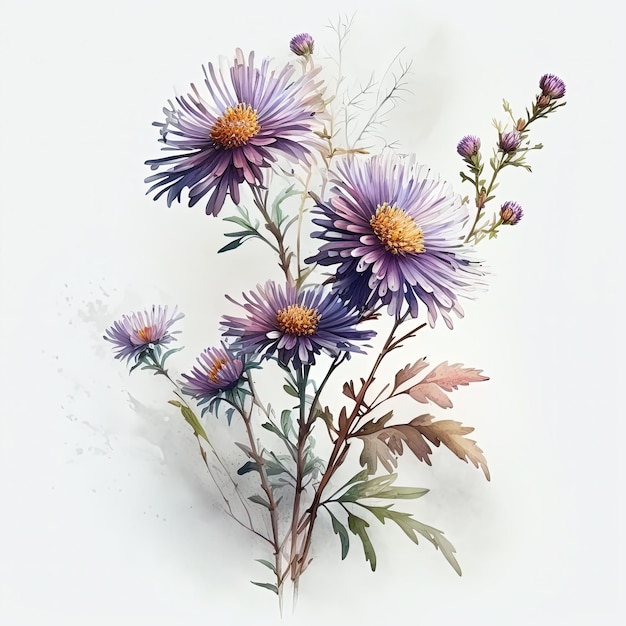This hyper-realistic illustration, set against a white background with a subtle hint of gray, showcases a strikingly detailed bundle of flowers. The flowers feature thin, pale lavender petals with hints of pinkish, whitish hues, in a graceful display of color gradation. At the center of each fully bloomed flower is a rich golden-yellow core, accented by tiny yellow-orange stamen. The image includes both fully opened blooms, numbering at least five, as well as about five buds that have yet to blossom. The flowers are supported by stems and branches that display a mix of green and brownish tones, interspersed with foliage in shades of green, bluish-green, light pink, reddish, and brown. This elegant composition, likely created with significant artistic skill, captures the intricate and delicate beauty of the subject matter, standing upright and vivid against the minimalist background.